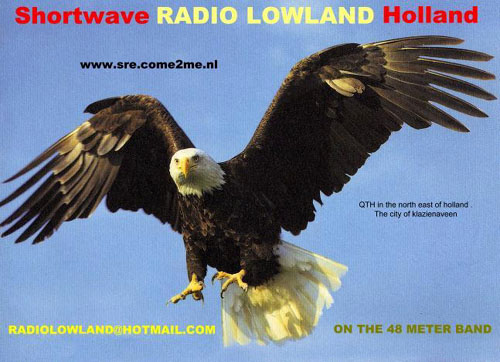The image depicts a majestic bald eagle flying against a light powder blue sky, with its large black wings partially outstretched, revealing a white head, white tail, and yellow beak. The eagle's sharp claws, yellow with black talons, are prominently positioned in front of it, as if poised to land or snatch prey.

At the top, the title "Shortwave Radio Lowland Holland" is prominently displayed, with "Shortwave" and "Holland" in capitalized red letters, and "Radio Lowland" in capitalized yellow letters. Just below the title, in smaller black text, is the URL: www.sre.com2me.nl.

Off to the right side of the eagle, it says "QTH in the northeast of Holland, the city of Klaasenaveen" in smaller black text. In the lower left corner, printed in all capitalized yellow letters, is the email address: RADIO LOWLAND@HOTMAIL.COM. On the lower right corner, in capitalized mustard green letters, it notes: ON THE 48 METER BAND.